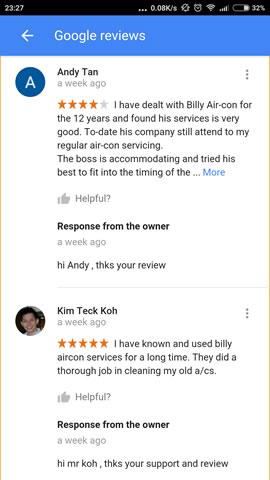In the image, a smartphone screen displays a Google search page at 23:27, with the status bar showing a 32% battery charge and active network bars. The prominent area features Google Reviews about "Billy Air Con," with notable contributions from users Andy Tan and Kim Tech Kong.

Andy Tan, in a blue circular profile icon with a white initial "A," posted a review a week ago, awarding four stars. His feedback highlights his 12 years of satisfactory service experience with Billy Air Con, especially appreciating the boss's efforts to accommodate scheduling.

Next, Kim Tech Kong, depicted in his profile image as an Asian man with black hair, gave a five-star rating. His review praises the meticulous cleaning of his older air conditioning units. Responses from the business owner are present beneath both reviews, expressing gratitude for their feedback.

The interface consists of primarily black, blue, and white colors, with accents of orange and thin lines of yellow enhancing the visual layout.